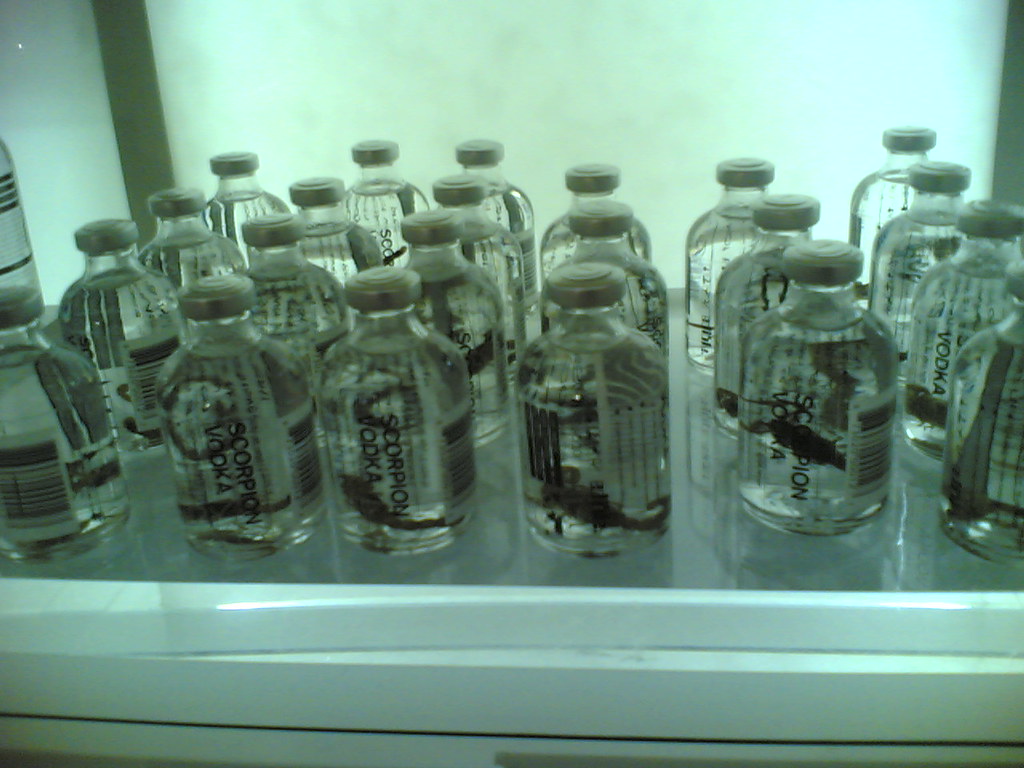This color photograph, taken in rectangular landscape orientation, exhibits a scene with a slightly off white balance, casting a faint greenish-blue tinge over the entire image. The main focus is a glass shelf adorned with numerous small, identical glass vials filled with a clear liquid. These vials, reminiscent of those used for medical injections, are topped with circular, grey metal caps and each bears a barcode on the side.

Upon closer inspection, when tilting the head 90 degrees clockwise, black vertical text reading “SCORPION” and horizontal text reading “VODKA” can be discerned on the bottles, suggesting that they contain an alcohol known as Scorpion Vodka. Despite their medicinal appearance, it is confirmed that they house a clear spirit, adding an element of surprise.

The vials are neatly arranged in six to seven rows, each row comprising six to seven bottles, all uniformly filled up to the shoulders just below the cap, with a slight air gap remaining. The shelf is situated in what appears to be an illuminated refrigerated cabinet, most likely in a medical, hospital, or doctor's office setting, given its white metal trim, glass top, and illuminated translucent back panel. The ambient lighting emanating from the cabinet and the unusual greenish hue contribute to the intriguing atmosphere of the image.